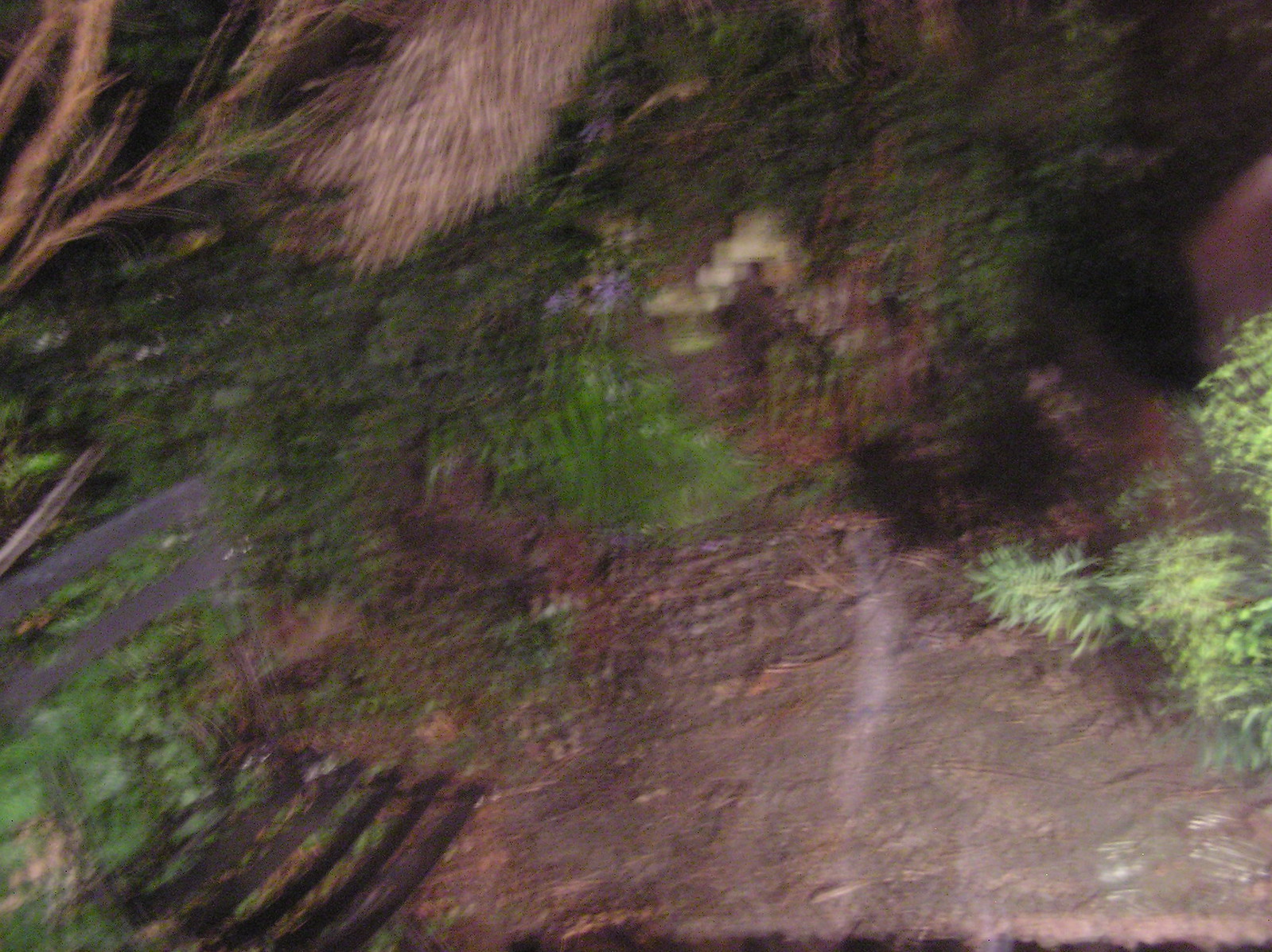The blurry nighttime photo predominantly features a dimly lit outdoor ground scene, likely illuminated by a flash or nearby light source such as car headlights. The ground comprises mainly dirt interspersed with some grass, twigs, and possibly leaf litter. To the left side, there's a black, flimsy-looking chair with thin horizontal slats on the seat and backrest, resting on the mixed terrain. A bush or ornamental grass, displaying various shades of green, can be observed on the right side of the image. Scattered around are indistinct elements that may include a rock, branches, and assorted debris. Additionally, an obscure object resembling a grid or crate sits among the greenery.